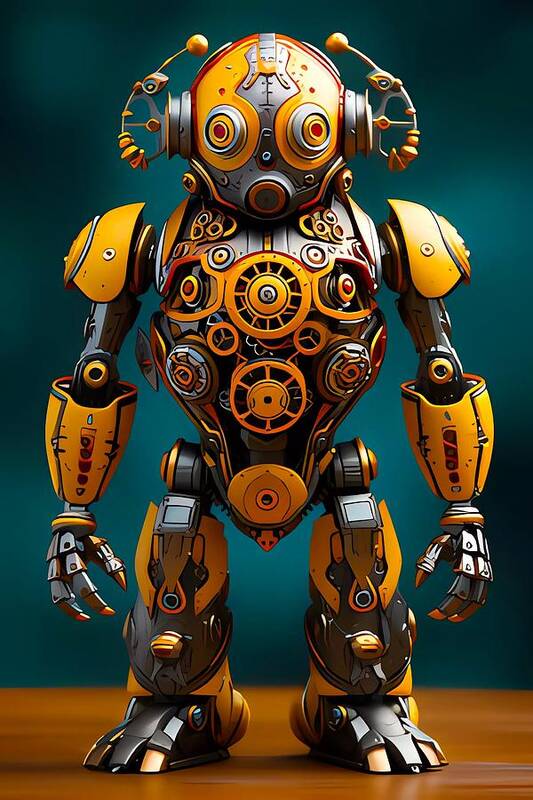The image showcases a detailed computer-generated illustration of a small robot standing on a wooden, yellowish-brown floor. The background transitions from this floor up to a dark green tone, with a lighter green halo surrounding the robot. The robot, which faces the camera with its arms resting by its sides, has a humanoid form with distinct robotic elements.

Its head is predominantly yellow, accentuated by silver and purple trim around its protruding silver eyes, which feature red centers. The mouth is a small yellow circle encircled by silver. The ears resemble handles with stems ending in ball-like structures, functioning as antennae. The robot's chest is decorated with an intricate array of yellow, red, and orange gears, topped with a silver chest plate.

The arms display a combination of mechanical and human-like characteristics: the shoulders are yellow, the biceps are silver, and the forearms are protected by large, round yellow plates, ending in silver hands with yellow-tipped fingers. The legs are similarly designed with yellow and silver segments, featuring significant protective guards running from the hips down to the feet, which are facing the camera and equipped with three silver toes each. The overall color scheme prominently features various shades of yellow and silver, giving the robot a striking and mechanical appearance.